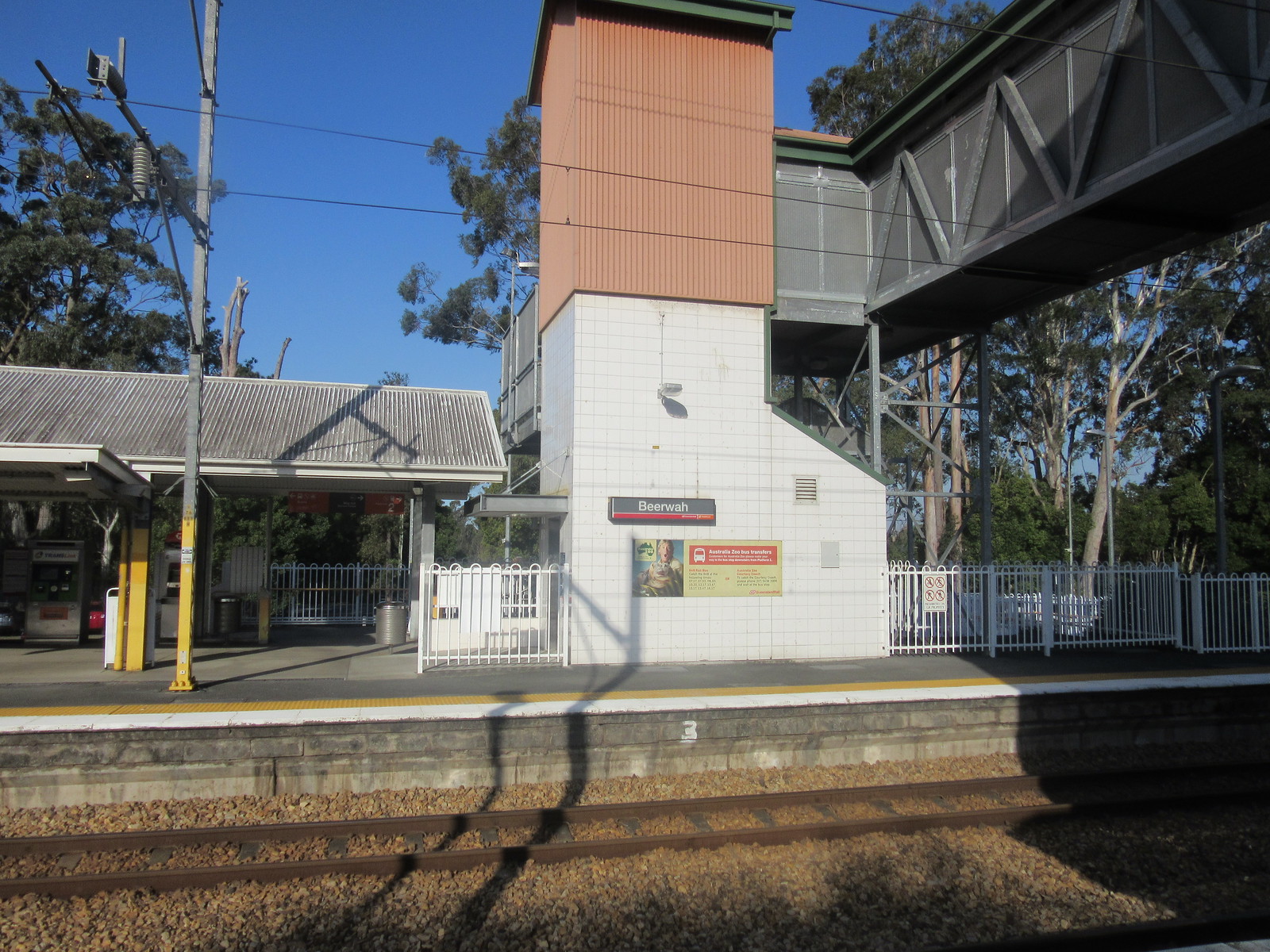The photograph captures a daytime scene at Beerwah train station, bathed in clear blue skies. The grey cement platform extends along the bottom of the image, with orderly tracks leading towards the horizon. A white metal fence encircles the station, with a gated entrance granting access to the platform. Above, an enclosed walkway bridges the tracks, leading to a stairwell that descends towards the platform and exits through the white gate. To the left, a sheltered waiting area with a greyish roof offers some respite, possibly housing ATMs for passenger use. A yellow-painted light pole stands as a solitary sentry amidst the serene emptiness. Prominently displayed is the station’s name “Beerwah” on a white wall, accompanied by a sign depicting Steve Irwin and a crocodile, advertising Australia Zoo and its bus transfers. Tall trees form a verdant backdrop, enhancing the tranquil ambiance of the deserted station.